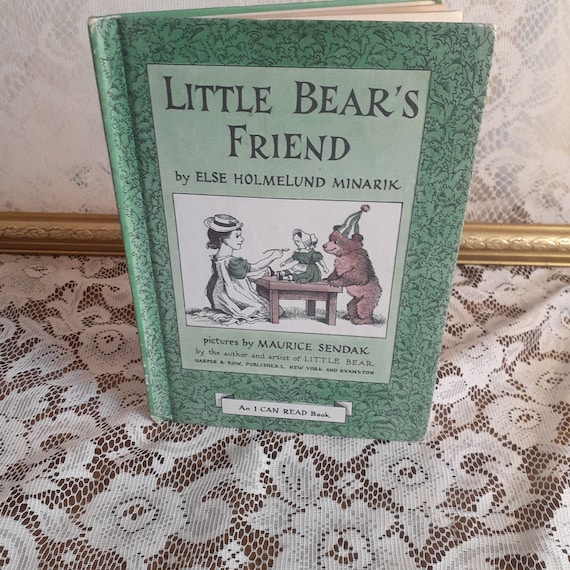In this square image, a book titled "Little Bear's Friend" stands upright on a lacy, white doily, which contrasts with the dark wood surface beneath it. The backdrop features a wall adorned with white floral or leaf-patterned wallpaper, and a strip of gold baseboard, possibly the bottom edge of a picture frame, runs horizontally behind the book. The book itself is green with a darker green pattern. At the top, the title "Little Bear's Friend" is prominently displayed, followed by "By Else Holmelund Minarik." Below this, it states "Pictures by Maurice Sendak," with some smaller, illegible print. An illustration on the book cover depicts a wooden table with a bear wearing a green and white striped hat standing to the right. A little girl in a white and green dress and a matching hat sits at the table, feeding a doll dressed similarly. The book is noted as "An I Can Read Book" at the bottom.